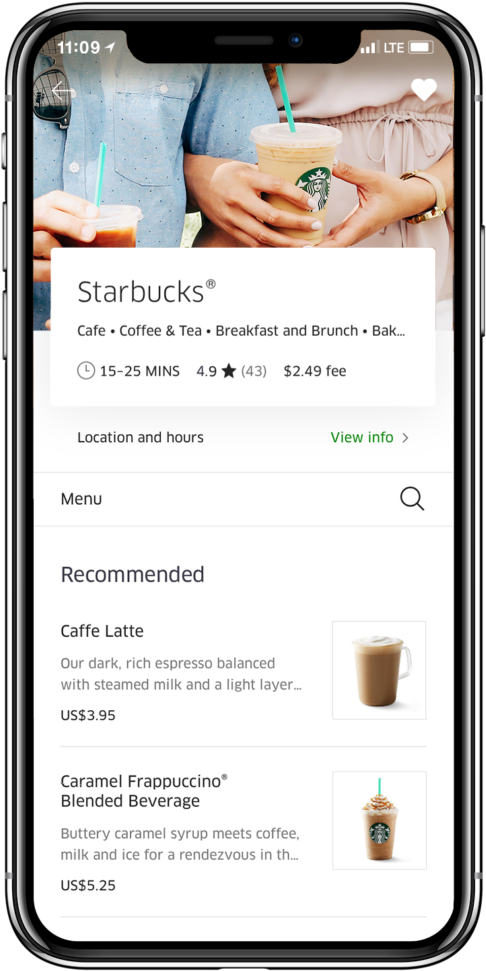This photograph showcases a sleek, black metal cell phone featuring prominent side buttons. The screen displays a digital time reading of 11:09 in the upper left corner, with indicators for cellular signal strength, LTE connectivity, a nearly full battery, and a white heart icon on the right.

The wallpaper is an intimate photo of a man and woman, captured from their chest area down to her waist. The man is dressed in a blue button-down shirt, while the woman sports a light pink, tan-colored outfit. Both are holding clear Starbucks cups displaying iced coffee and green straws. 

Centered at the bottom of the screen is a detailed description of a local Starbucks café, including its offerings and reviews. The text highlights "Starbucks cafe coffee and tea breakfast and brunch" followed by "BAK..." indicating a truncated location name. It mentions an estimated delivery time of "15 to 20 minutes," a rating of "4.9 stars" from "43 reviews," and a delivery fee of "$2.49." Below, "location and hours view info" is highlighted in green. Menu recommendations include:

1. **Cafe Latte**: "Our dark rich espresso balanced with steamed milk and a light layer..."
   - Price: "$3.33 USD"
   
2. **Cream Caramel Frappuccino Blended Beverage** (noting Frappuccino is a registered trademark): "Buttery caramel syrup meets coffee, milk, and ice for a rendezvous in the..."
   - Price: "$5.25 USD"